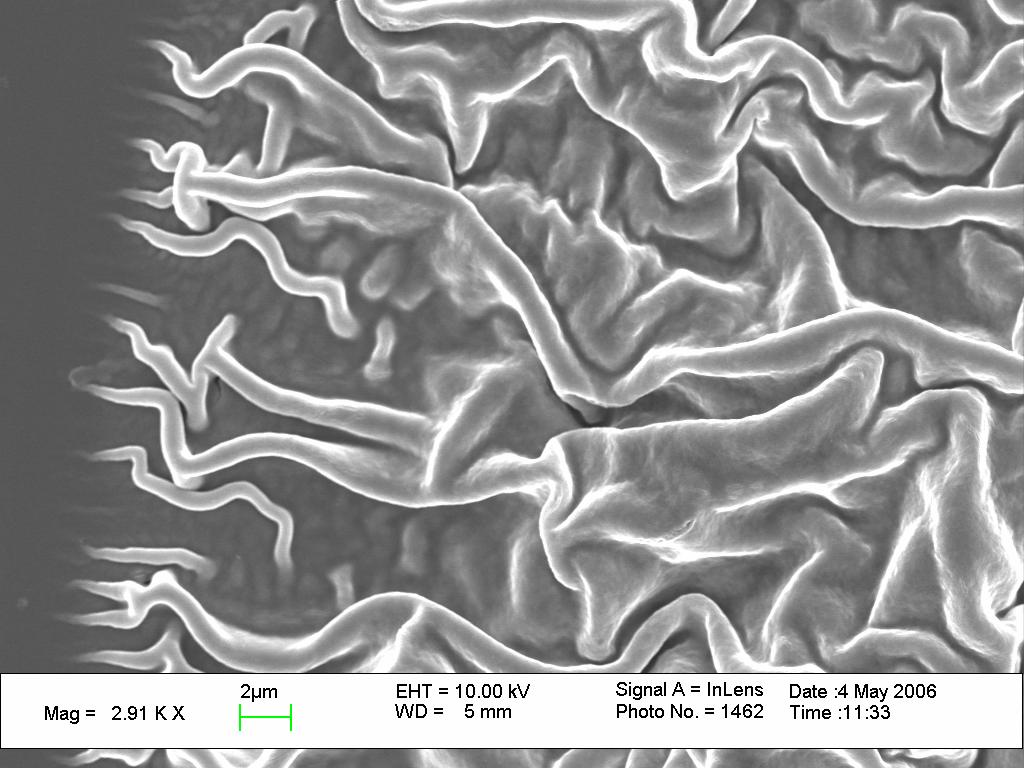The black-and-white photograph appears to depict a highly magnified microscopic organism, possibly captured using an electron microscope. The central focus of the image resembles the intricate, wrinkled textures akin to folds of cloth or brain tissue, rendered in grayscale. The photograph has dimensions of approximately five by five inches. Along the bottom of the image, there is a white strip containing several scientific annotations in black text. From left to right, the information reads: "MAG = 2.91 KX," followed by a green measurement marker indicating "2 μm" (micrometers). Further to the right, it states "EHT = 10.00 kV," "WD = 5 mm," and "Signal A = InLens." The identification number of the photograph is "Photo No. 1462." Additionally, it provides the date "4 May 2006" and the time "11:33," although it does not specify a.m. or p.m. The entire image, including the annotation strip, is enclosed within a thin black border.